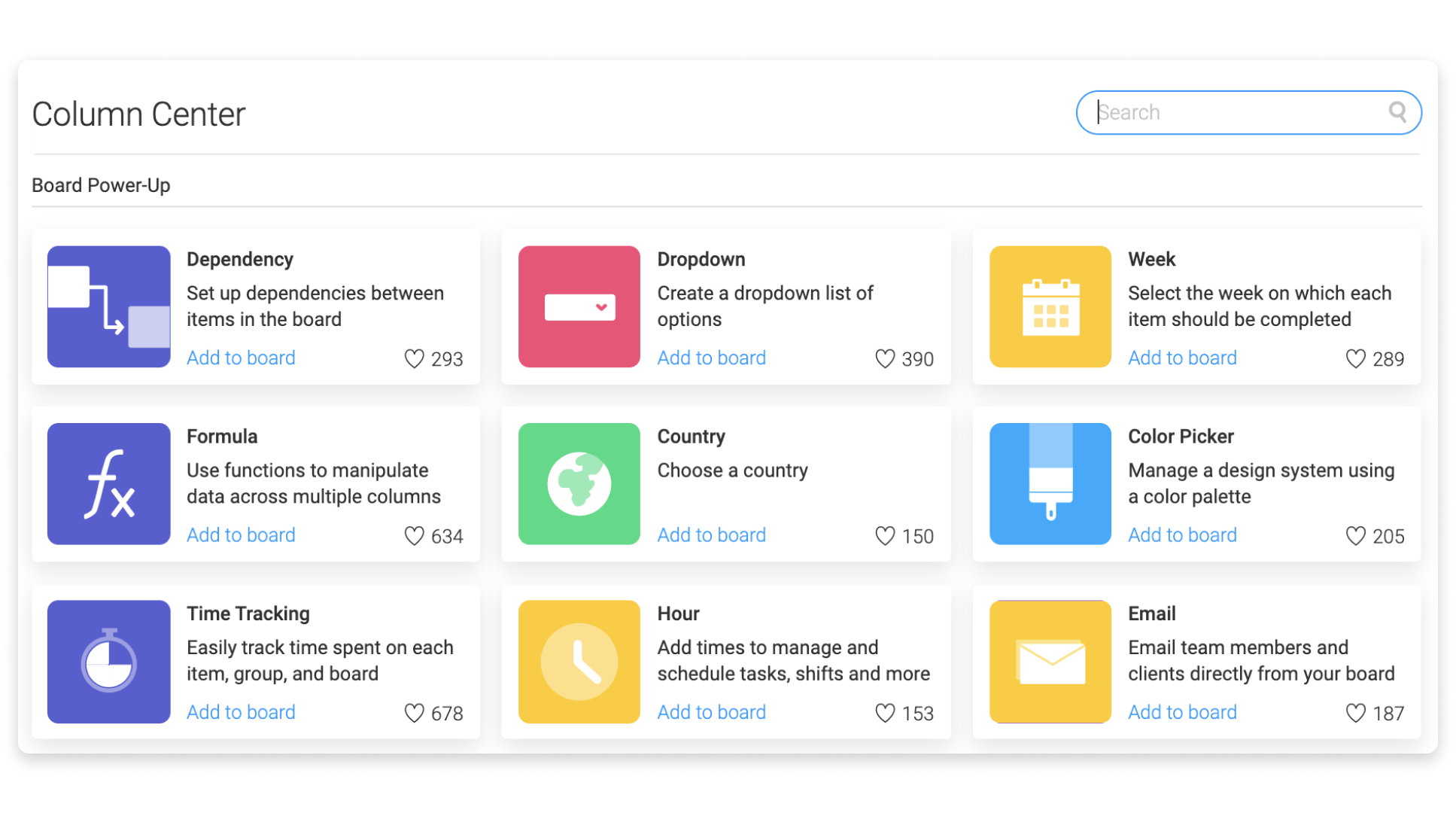The image consists of several colored and outlined sections arranged in a grid-like layout. 

- **Top Section**:
  - A gray-outlined rectangle has a label on the top left corner that reads "Column Center". Below this label, a thin gray line spans across the section.
  - On the right side of this top section, there is a blue-outlined rectangle that bulges out at the sides with the word "Search" and a magnifying glass icon.

- **Middle Section**:
  - Immediately below the thin gray line, on the left, the text "Word Power Up" is displayed. 
  - Another gray line is located beneath this text.
  - Under the second gray line, there is a white rectangle featuring a purple image, surrounded by text in both black and blue, and a heart icon followed by a number.
  - Adjacent to this, another white rectangle includes a blue square with "FX" written inside. It also contains text in black and blue, a heart with a number, and a purple square with a timer clock icon.

- **Following Rows**:
  - Proceeding to the right of these white rectangles:
    - A pinkish-red square has a white rectangle inside, and accompanying text in black and blue, along with a heart and a number.
    - Next, a green square presents a globe icon and contains similar text formatting, a heart, and a number.
    - A yellow square showcases a lighter yellow circle depicting a clock, with words in black and blue, a heart, and a number.
  - In the final row:
    - An orangey-yellow square features a calendar icon with text in black and blue, a heart, and a number.
    - A blue square houses a paintbrush icon, trailing a lighter blue swath, and includes words in black and blue, a heart, and a number.
    - Lastly, a yellowy orange square displays a white envelope icon, accompanied by black and blue text, a heart, and a number.

This grid layout is color-coded and includes icons representing various functionalities or categories alongside descriptive text, hearts indicating likes or favorites, and numerical values.